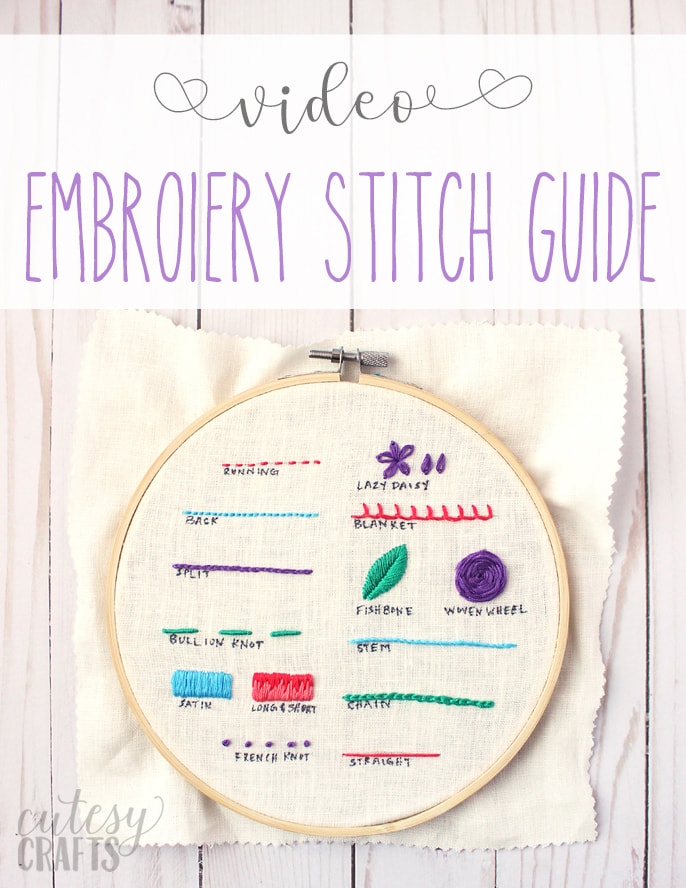This screen capture is from a video titled "Video Embroidery Stitch Guide," though there's a typo in the word "Embroidery" (spelled "Embroiery") on a white banner at the top. The word "Video" is presented in fancy gray script on a translucent black background, while "Embroidery Stitch Guide" appears in bold, all-capital purple letters. The main focus of the image is an embroidery hoop placed on a whitewashed wooden plank table. Inside the hoop, various sample stitches are displayed in vivid colors: lazy daisy in purple, blanket stitch in red, back stitch in light blue, split stitch in purple, and stem stitch in light blue, among others. Each type of stitch is clearly labeled in black, which is embroidered directly onto the fabric. At the bottom left corner of the frame, the video source is identified as "Cutesy Crafts," with "Cutesy" in script and "Crafts" in all caps and faded gray font. The fabric extends out of the embroidery hoop and partially covers the wooden background, showcasing a neatly organized array of stitching styles in hues of purple, aqua, red, and green.